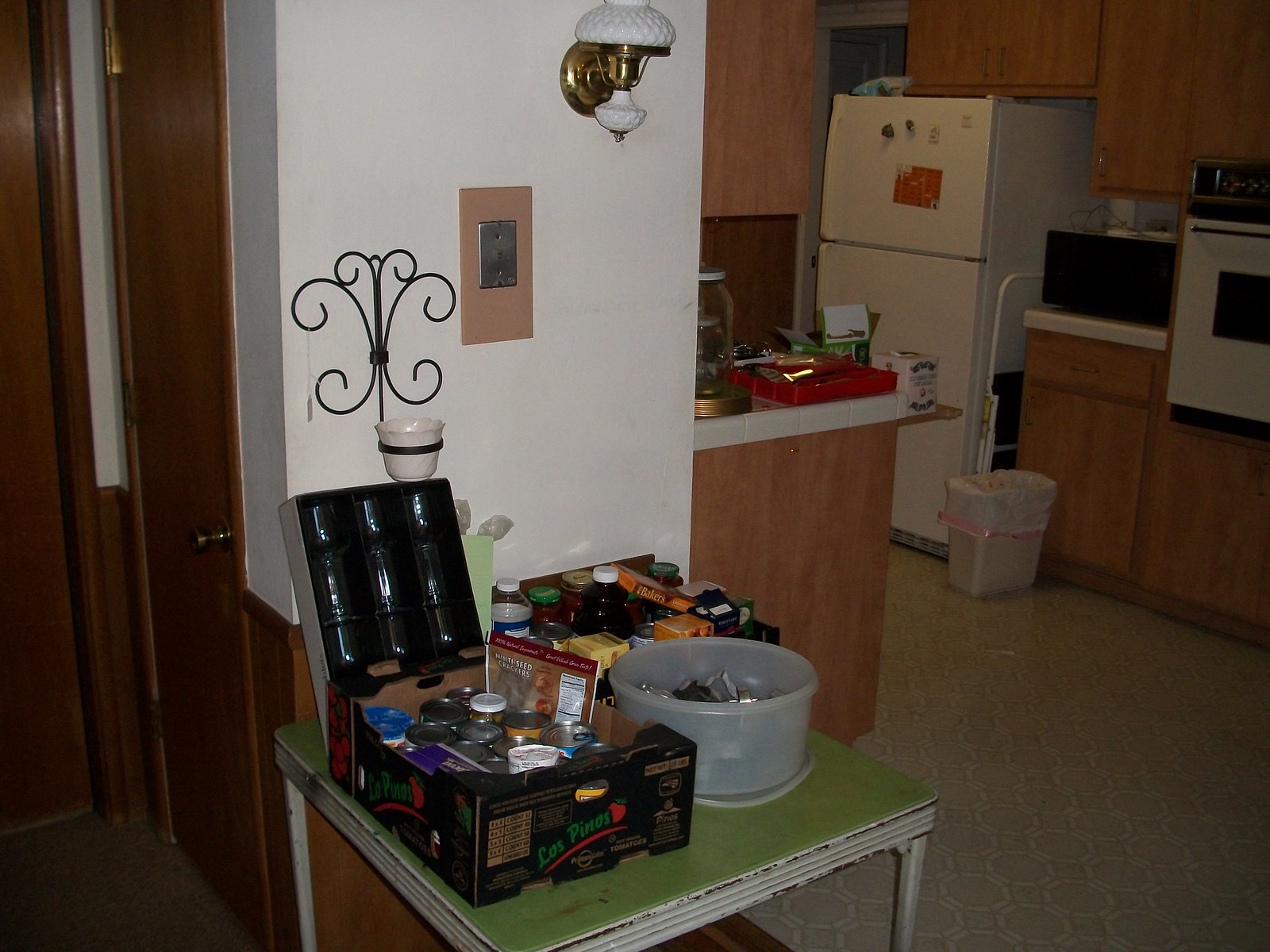The photograph captures the interior of a residence with a central focus on a table that resembles the size of a card table. The table features silvery metal legs and trim, both heavily corroded. The tabletop, colored green, appears corroded or dirty. Atop this table sits a large, translucent container filled with shiny metal objects, under which the container's lid lies. Besides the container, there's a large wooden box, black on the outside, adorned with various writings and drawings. The green lettering reads "Los Pinos" with a depiction of a red tomato and white lettering faintly indicating "tomatoes". Inside the box are an assortment of jars and unopened cans; the jar lids vary in color, some white, others black. Additionally, a labeled bag of what seems to be multi-seed crackers rests on the table.

Against the wall, there's a large black box containing shiny, reflective objects whose material—glass or metal—remains unclear. The wall itself is white. Mounted above the box is a wrought iron filigree decoration holding an empty vase. Adjacent to this décor is a corroded chrome light switch with a tan surround. Further up, there's a light fixture combining a brass base with a milk glass lampshade, featuring brass accents as well.

To the left, a wooden door with a brass-colored doorknob opens, and a dark brown floor is visible. The right side of the table transitions into a kitchen area featuring a light tan linoleum floor. A white waste paper basket stands next to a white refrigerator, positioned before wooden counters. An oven is mounted in the wall, framed by brown cabinets above it. The kitchen space further includes a small wooden counter with an indistinct black object on it. The walls display a wood grain pattern, light on the upper half and darker on the lower half, and a white tiled countertop behind holds indistinguishable objects due to the photograph’s blurry quality.